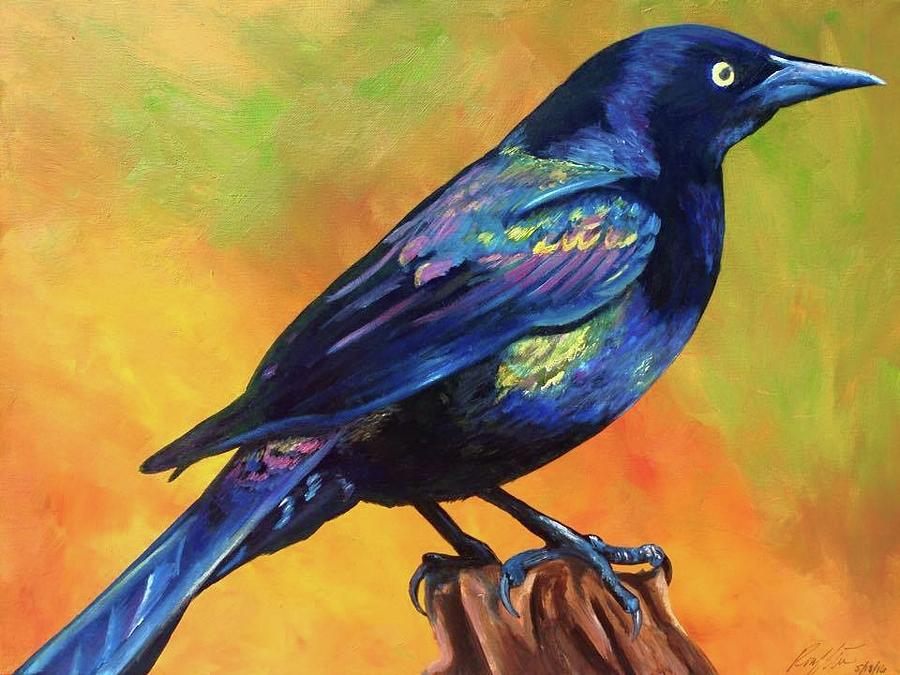This rectangular painting captures a solitary blue European starling perched serenely on a wooden stump. The bird, predominantly a dark indigo-blue, stands out with its iridescent feathers that shimmer with hints of yellow, deep red, and lighter blue, especially noticeable on its wings, belly, and tail. The bird's pointy beak and striking yellow eye with an offset black pupil draw the viewer's attention. It remains motionless, facing right, highlighted by its long nails gripping the stump. The background is a vibrant abstract mix of oranges, yellows, and greens, rendered in soft, uneven brushstrokes that evoke a warm, almost ethereal atmosphere. The artist's signature can be seen in the bottom right-hand corner, though slightly obscured.